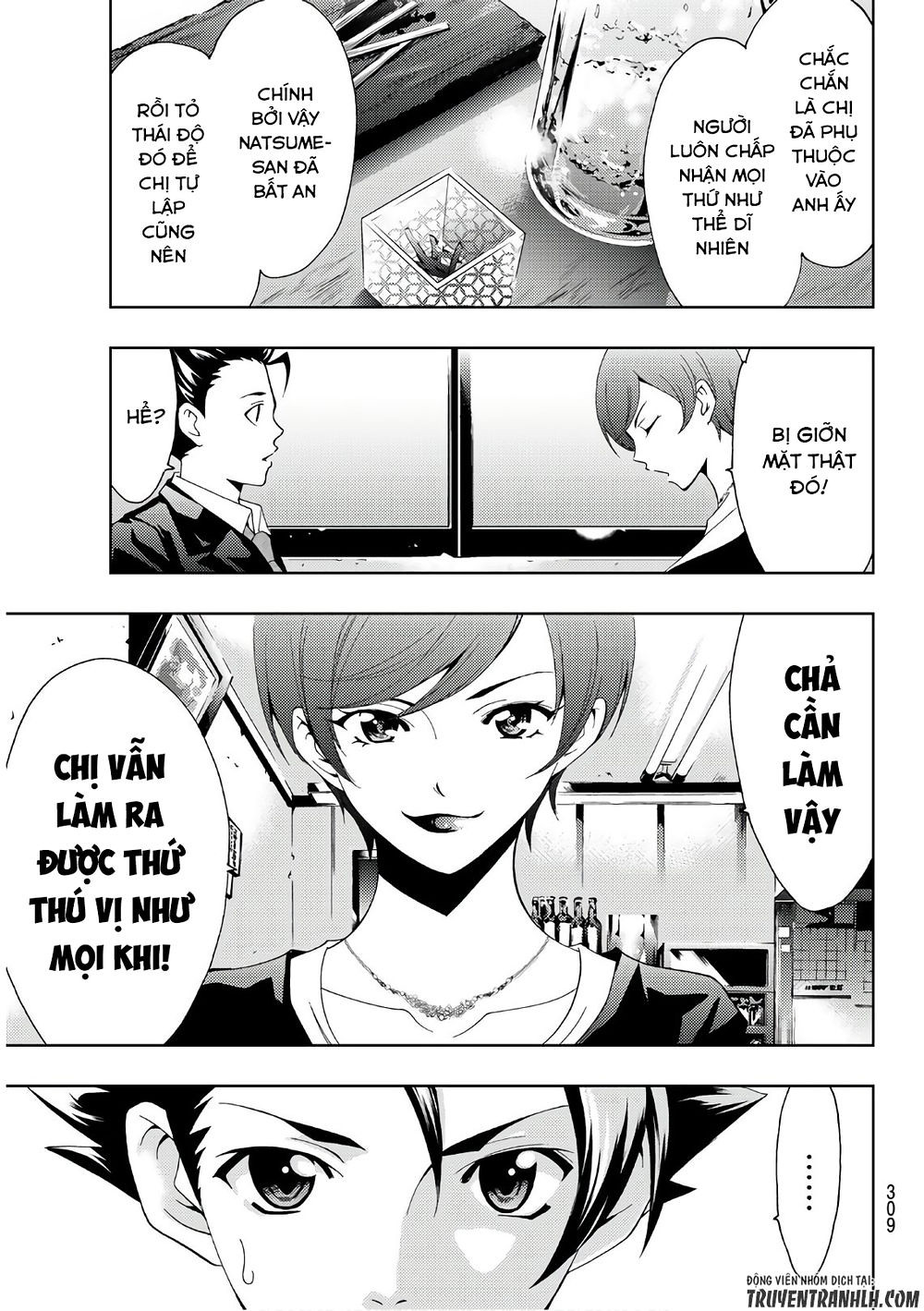The image is a black-and-white comic strip page, divided into four horizontal sections. The comic is presented in a Japanese anime style with serious expressions on the characters' faces, and the dialogue is in Vietnamese, which adds a layer of intrigue and cultural specificity. 

In the top strip, we see a tabletop adorned with a bottle and some matches, setting a somewhat domestic or casual scene. The second strip below centers on a wall, with two characters positioned on either side—one to the right and one to the left—engaging in a conversation. Both are depicted from the shoulders up, facing each other. 

The third strip features a frontal view of a woman, shown from the shoulders up. Behind her left shoulder are some bottles, while behind her right shoulder is a wall possibly decorated with pictures. This detail adds depth to the setting, suggesting a room or a bar-like environment. 

The bottom strip displays a close-up of a person's face, cropped just below the eyes, emphasizing their intense, possibly emotional expression. 

At the very bottom right of the page, a website URL, "trueventronnlh.com," is prominently displayed, indicating a Vietnamese site that could provide further context or continuation of the comic.

This detailed depiction not only describes the visual arrangement but also hints at the narrative and emotional tone of the comic.